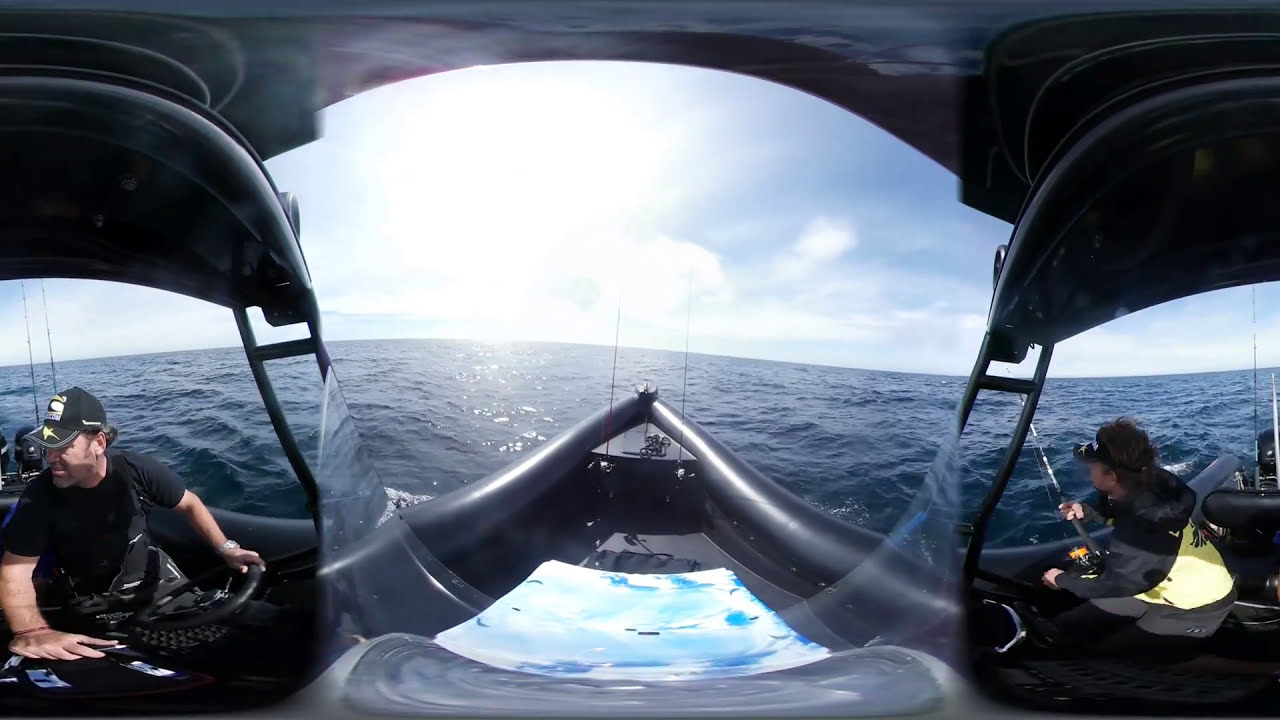The image showcases a 360-degree panoramic view taken from inside a pontoon-like boat navigating the middle of the ocean. The deep blue water exhibits noticeable waves and a slight choppiness, indicating a lively sea. The sky above is a clear blue, interspersed with sparse white clouds, and the sun shines brightly, casting a strong illumination across the scene.

On the left side of the boat, a man stands at the steering wheel, wearing a black short-sleeve shirt and a black baseball cap adorned with some lettering. His hands grip the wheel as he gazes over his right shoulder. Towards the far right of the image, another individual, donned in a black hooded jacket with a yellow band around the middle, sits at the edge of the boat. This person, who has brown hair, is holding a fishing rod, poised to fish in the surrounding waters. Multiple fishing rods are also visible, positioned along the boat's edge, adding to the scene's recreational ambiance.

The boat's interior and its top surface are black, with a framework supporting the overhead covering, which is shadowed against the vibrant backdrop. Together, these elements combine to provide a vivid and comprehensive depiction of a sunny day spent fishing on a lively ocean.